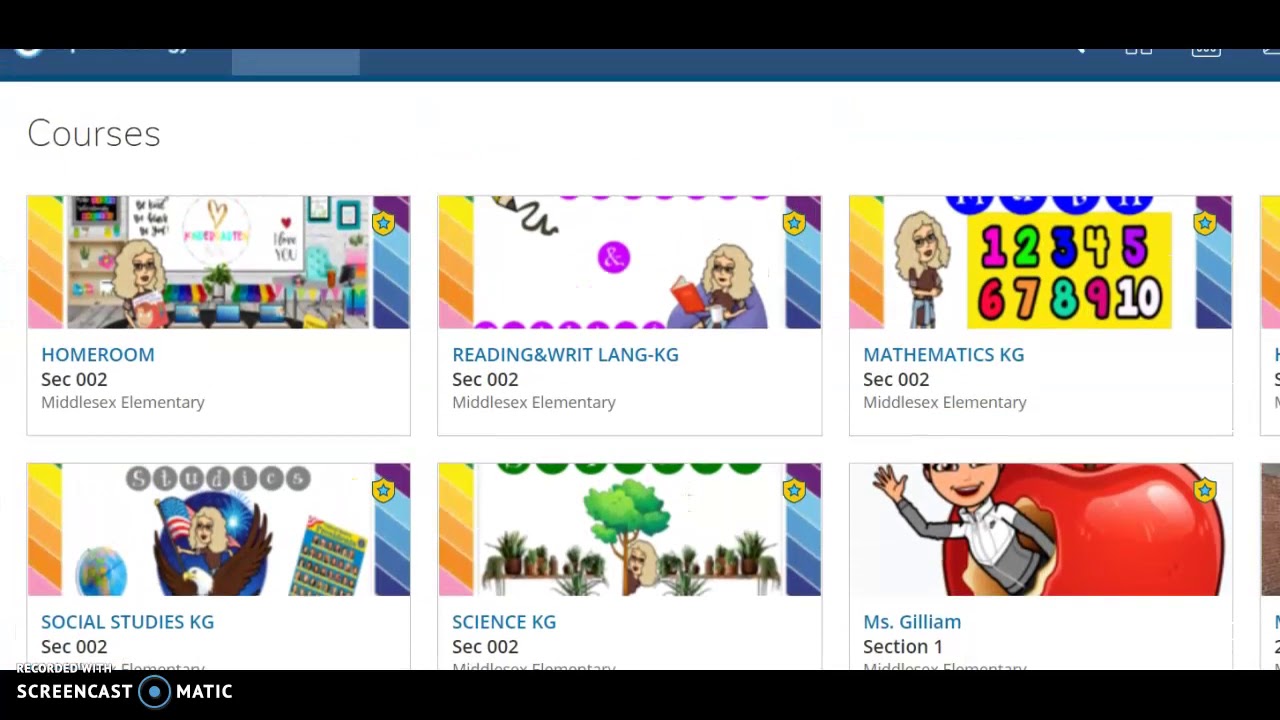The image depicts a partially visible computer screen, predominantly focused on an educational dashboard with various course offerings. At the top, there is a black banner, and beneath it, a dark blue banner that is partially cut off. The main section of the screen is white and features the word "Courses" prominently on the left-hand side.

Six course tiles are visible, arranged in two rows of three, with additional course tiles partially visible on the right-hand side. The first course tile is labeled "Homeroom sec002 Middlesex Elementary" and includes a cartoon avatar of a blonde-haired woman with glasses, resembling a teacher. The second tile, "Reading and Writing Language-KG sec002 Middlesex Elementary," displays the same cartoon teacher figure, this time depicted reading a book. The third tile is titled "Mathematics KG sec002 Middlesex Elementary."

The bottom row features the following courses: "Social Studies KG," "Science KG," and "Miss Gilliam section 1," which is different from the previous course titles. 

The screenshot appears to have been captured using Screencast-O-Matic, as noted at the bottom of the image. This likely indicates that the screen shows a collection of educational resources or lesson plans created by a teacher for various kindergarten courses at Middlesex Elementary.